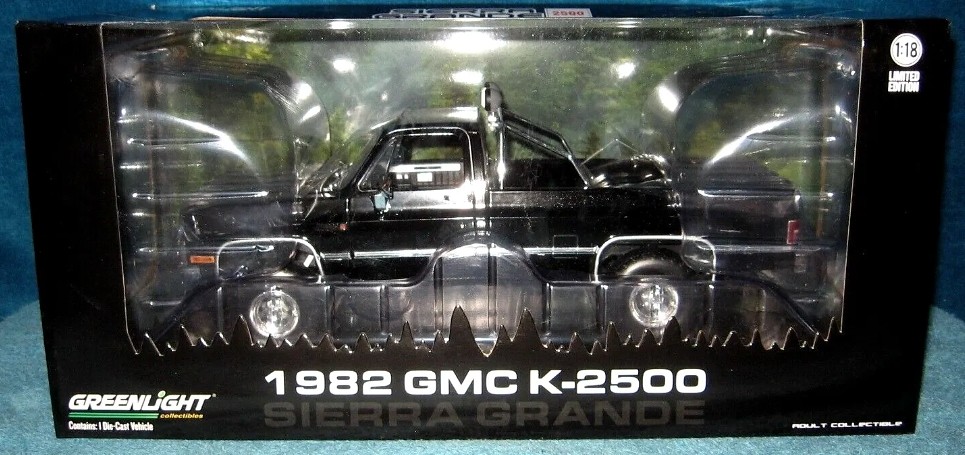The image features a meticulously detailed model of a 1982 GMC K2500, still securely housed within its original packaging. This model, designed as a toy yet sophisticated enough for adult collectors, is a limited edition piece produced by GreenLight Collectibles. The die-cast vehicle, resplendent in a sleek black finish, is showcased prominently through the clear display window. The box, similarly black with contrasting white text, denotes significant details including the 1:18 scale of the model, emphasizing its precision and authenticity. Positioned on a blue table, the box presents a striking juxtaposition, further highlighting the model’s intricate design and collectible status.